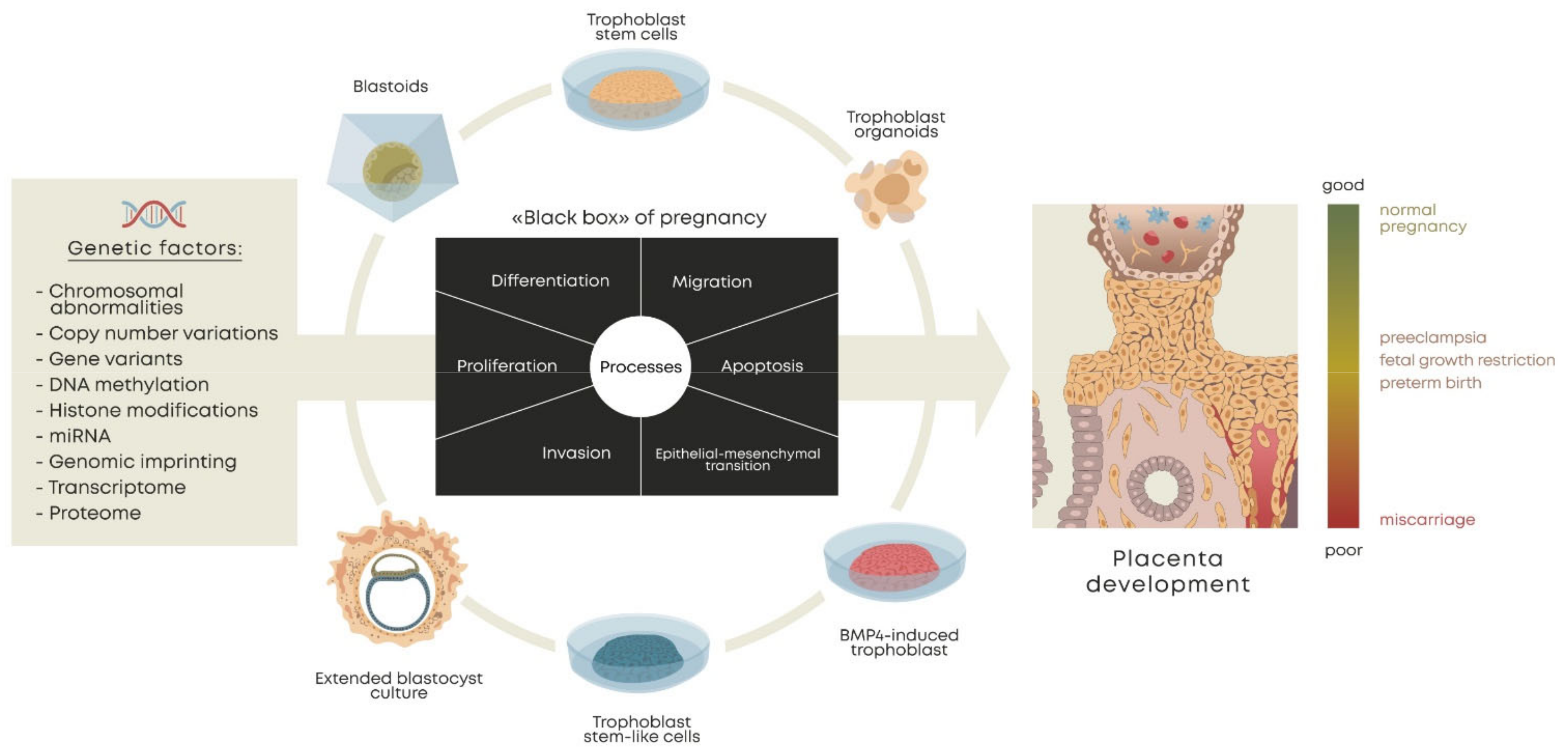This detailed educational medical chart illustrates the various phases and genetic factors impacting pregnancy outcomes. On the far left, there is a beige box labeled "Genetic Factors," listing critical elements such as chromosomal abnormalities, copy number variations, gene variants, DNA methylation, histone modifications, miRNA, genomic imprinting, transcriptome, and proteome. An arrow from this box leads to a central circular diagram surrounded by smaller images representing blastoids, trophoblast stem cells, trophoblast organoids, BMP4-induced trophoblast, trophoblast stem-like cells, and extended blastocyst culture. These smaller images each feature illustrative icons. At the core of the circle is a black rectangle known as the "black box of pregnancy," which identifies key processes including differentiation, migration, apoptosis, epithelial-mesenchymal transition, invasion, and proliferation. This arrow continues towards the right, connecting to an image labeled "placenta development." Adjacent to this image is a gradient bar transitioning from red at the bottom (labeled "poor") to green at the top (labeled "good"). Accompanying this gradient are different pregnancy outcomes: "miscarriage" in the red zone, "preeclampsia, fetal growth restriction, and preterm birth" in the middle yellow zone, and "normal pregnancy" in the green zone. This chart thoroughly details how genetic factors influence the developmental processes and potential health outcomes of pregnancy.